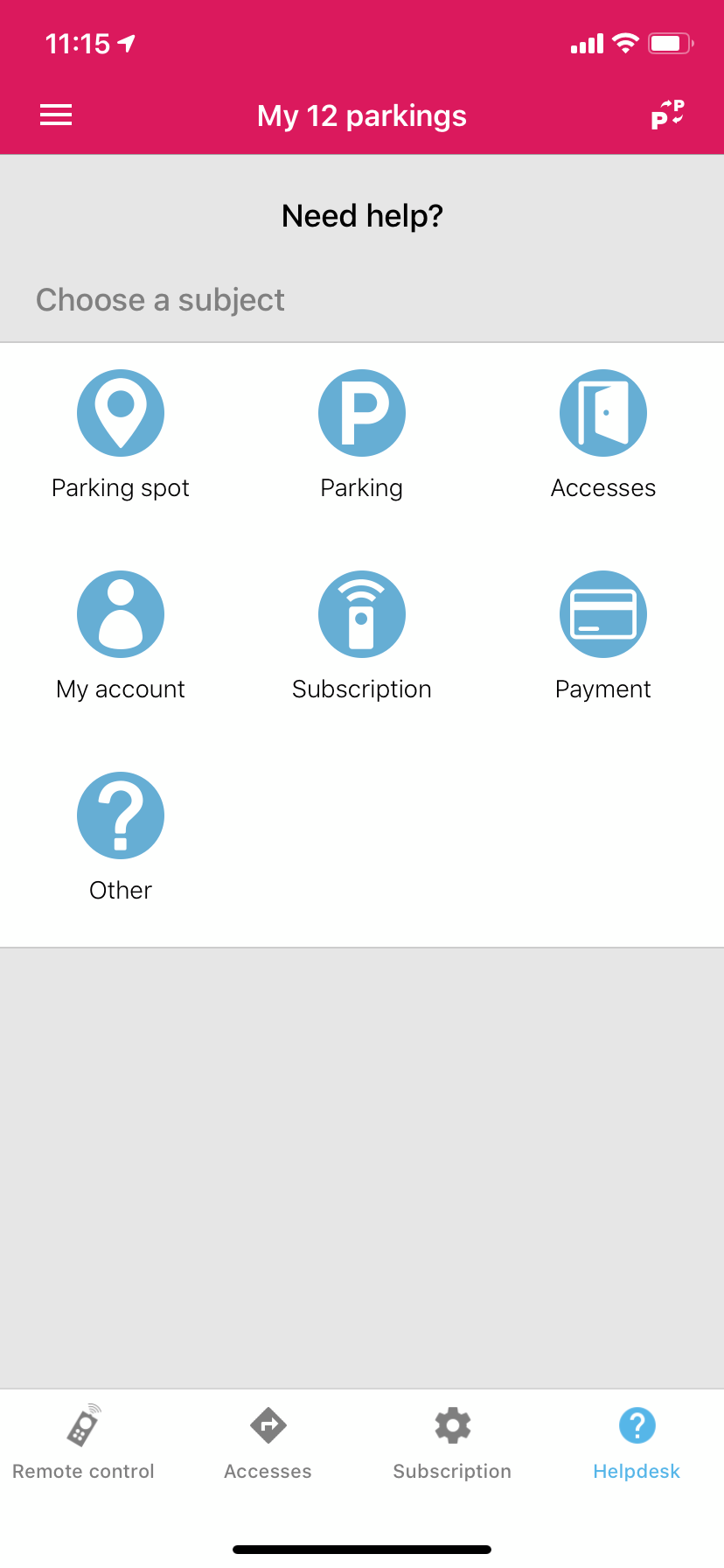The screenshot captured on a cell phone illustrates a mobile app interface with a plethora of details. At the top, typical status indicators are clearly visible: the time is 11:15, there are indicators for signal strength and Wi-Fi connection, and the battery level is displayed. All status indicators are rendered in white text against a red background. 

Beneath these elements, the red background continues with additional white text. On the far left, there is a menu bar icon. The title "My 12 Parkings" is prominently displayed in the center, while to its right is a 'P' symbol, likely referencing parking records.

Further down, a gray bar labeled "Need Help" appears, with subsequent text stating "Choose a subject." Below this gray bar is a section with a white background, hosting seven distinct icons arranged in two rows:

1. **Location Icon in a Circle:** Labeled "Parking Spot"
2. **Capital 'P' in a Circle:** Labeled "Parking"
3. **Open Door Icon in a Circle:** Labeled "Accesses"
4. **Outline of a Person in a Blue Circle:** Labeled "My Account"
5. **Phone with Signal Bars Icon:** Labeled "Subscription"
6. **Credit Card Icon in a Blue Circle:** Labeled "Payment"
7. **Question Mark in a Blue Circle:** Labeled "Other"

At the bottom of the screen, there is a large gray box occupying about a third of the display, which remains empty. Below this gray box are several icons featuring labels such as "Remote Control," "Accesses," "Subscriptions," and "Helpdesk."